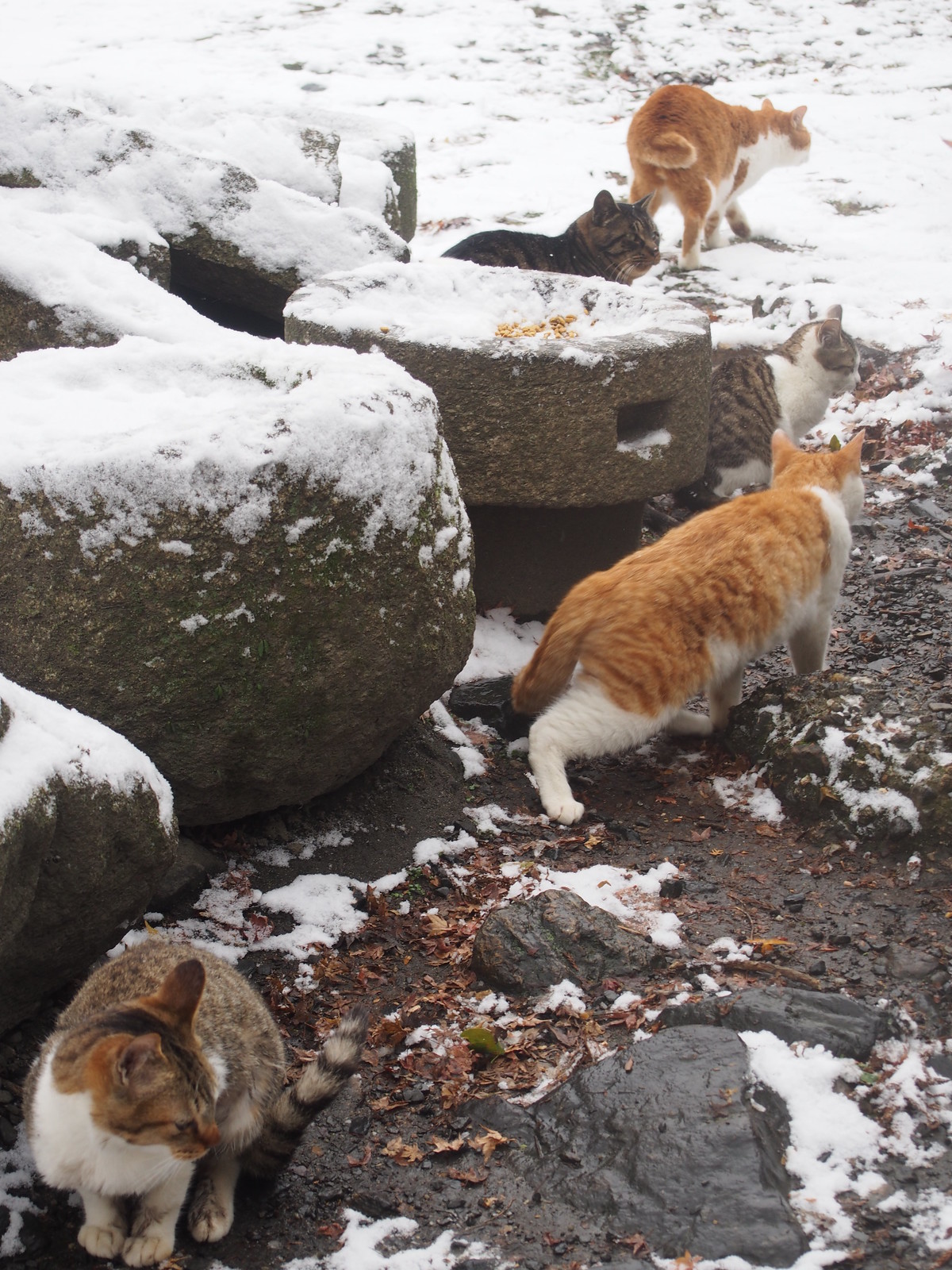In this snowy outdoor landscape, a group of five diverse cats is gathered near three large, snow-capped boulders on the left side of the image. The foreground features a brown and white cat with a striped tail sitting near one of the snow-covered stones, its front paws tucked in. Nearby, an orange and white cat appears to be walking away towards the top right. Surrounding these cats, patches of mud and small snow-covered stones create a textured ground. Further back, three more cats are clustered together, all facing in the same direction. These include another brown and white cat, a dark brown one, and a cat with an orange body and white underbelly. Each cat's unique color pattern contrasts vividly against the frosty backdrop, highlighting the serene and cold atmosphere of the scene.